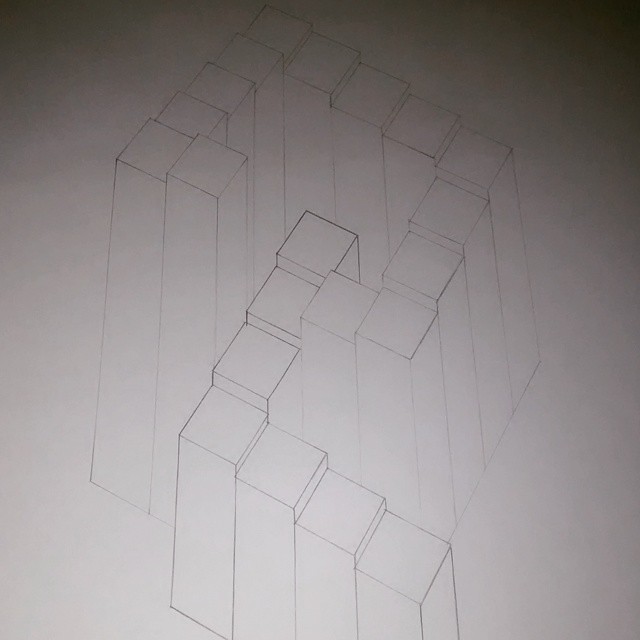The image showcases a detailed pencil drawing on a white piece of paper, depicting a three-dimensional shape composed of tall rectangular pillars with square tops. These pillars create a pathway-like structure that begins at the bottom middle of the image and ascends at an angle. The pathway turns right, continuing upward toward the top of the page, then shifts right again, heads upward, and veers to the left before descending and moving horizontally. The drawing employs shading techniques to enhance depth, with the tops of the pillars darkened to accentuate their 3D effect. The image is captured from a top-down perspective, and lighting variations make the upper part appear darker than the bottom, suggesting indoor photography. Despite its intricate layout, the depicted shape does not form any recognizable pattern, adding an abstract quality to the artwork.